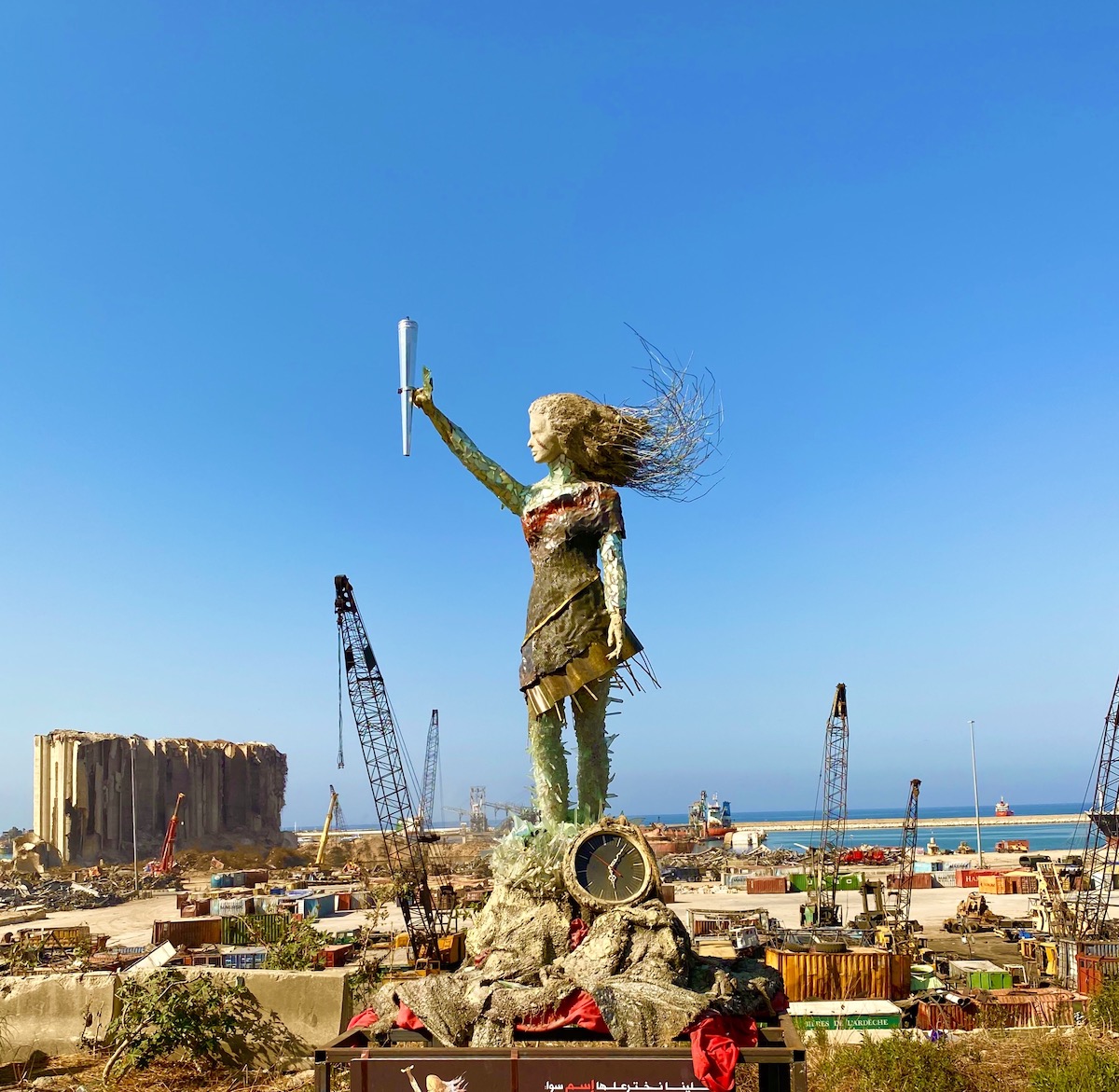In this daytime outdoor photograph, we are shown a striking statue of a young woman standing amid an industrial area, likely a shipping port, bordered by a large waterway under a clear blue sky. The background is filled with heavy machinery and cranes—up to five in the image—indicative of the site's function of lifting and transporting large items. The statue, which appears to convey a sense of motion and energy, features the woman holding a handle-like object overhead with her right hand, reminiscent of a torch, while her left hand rests by her side.

The woman's hair cascades dynamically behind her, and she is adorned in attire that seems pieced together from various materials, resembling scraps or street art, enhancing an impression of resilience. Her dress drapes over one shoulder, with a red trim and visible wire framing that hints at its construction. Her legs and arm are crafted from a green-bronze material, embellished with scale-like and fin-like details.

Standing on a rocky base, the statue is anchored by large concrete blocks and features a clock showing the time around 6.05, suggesting late afternoon. The area surrounding the statue is dotted with what seems to be shipping canisters and damaged containers, further adding to the rugged, industrial aesthetic. A buoy floating in the distant water reinforces the maritime context, and a few pieces of bush and a vertical rock formation are visible in the composition, adding to the textured and intricate setting.